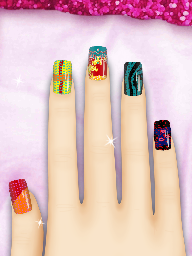This color photograph appears to be a digitally manipulated image, possibly created using Photoshop, showcasing a pale mannequin or artificial hand with long, slender fingers extending upward from the bottom portion of the image. Each fingernail features a unique, brightly colored design, resembling an advertisement for stick-on nails. The thumb nail is a vibrant magenta orange, while the index finger displays a green base with an orange cross. The middle finger nail has a gold and red bottom transitioning to a cyan or aqua top. The ring finger boasts a dark blue and black swirl pattern, and the pinky nail is adorned with a metallic pink and purple hue. The image is set against an indistinguishable background that might be fabric, stone, or another surface, partially covered with white cotton-like material. Above the hand, the upper section of the image is accented with bright pink glitter, adding a touch of sparkle that complements the colorful, rectangular-shaped nails.